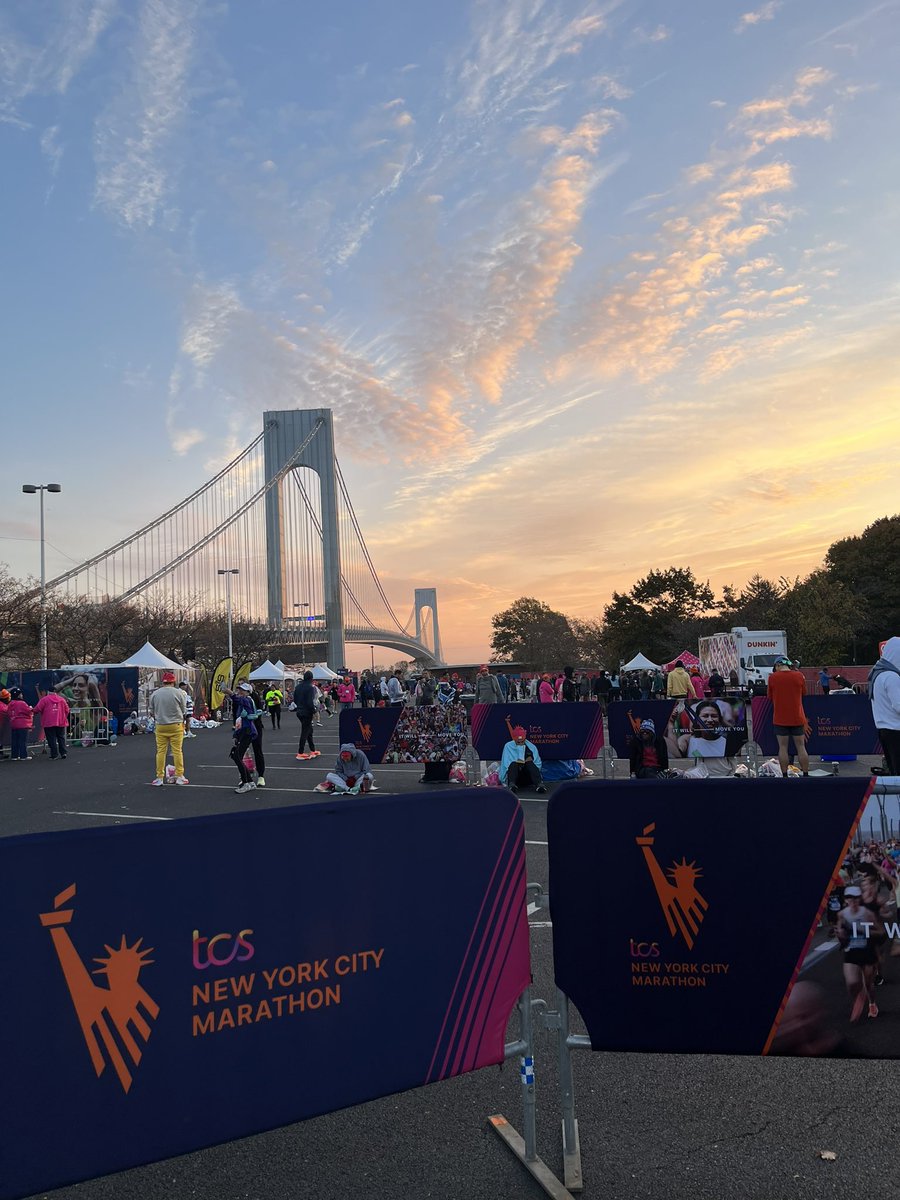The image depicts the starting area of the TCS New York City Marathon on an early morning. In the foreground, there are dividers with a blue background and pink stripes in the corners that display "TCS New York City Marathon" alongside a stylized orange Statue of Liberty logo. On the right side, another banner contains photos and text, although they are not fully legible. Multiple barriers of both styles can be seen extending into the background.

Participants are scattered throughout a large, dark gray asphalt parking lot, marked with white parking lanes, and many are sitting on the ground waiting for the race to begin. Spectators along the sidelines are dressed in brightly colored outfits, including pink, as well as hats, long-sleeved shirts, and various colored pants like black, gray, and yellow. 

The scene includes pavilions set up on either side of the fairway and small booths with people milling around. A distinctive Dunkin' Donuts truck is parked on the right-hand side. In the background, one of Manhattan's suspension bridges is visible, characterized by its gray concrete columns and steel cables.

The sky above is a mix of blue with white clouds, and the sun appears to be either rising or setting, casting a yellowish hue through the clouds. There is also a tree line with green leaves and some bare trees to the left, enhancing the vibrant yet tranquil atmosphere of the event's commencement area.